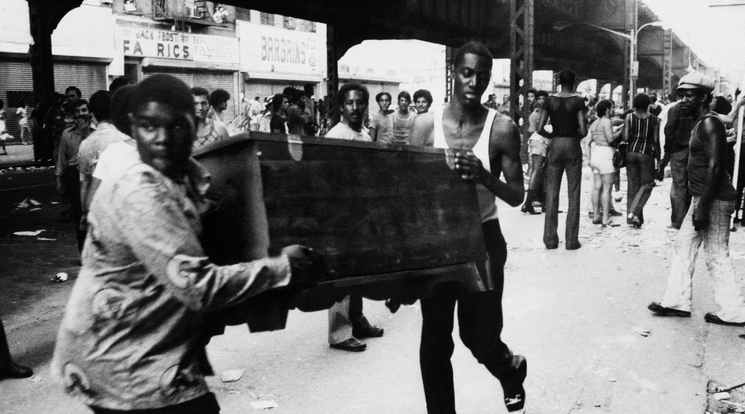This historical black-and-white photograph, likely from the 1960s or 70s, features a bustling street scene with African-American individuals, perhaps in the U.S. The image is horizontally aligned and shows an older street with an elevated bridge or railroad in the background. On the left side across the street, there are several shops with partially visible signs—one advertises "fabrics" (missing the 'B') and another "bargains."

The focal point of the photo is two men carrying a large, dark wooden piece of furniture; one is walking backwards, appearing to struggle, while the other walks forward. Their attire reflects the era, with one man notably wearing white bell-bottom pants, a tank top, and a floppy hat. Surrounding them are onlookers, suggesting that this might be a scene from a demonstration or event. The street is lively with people either standing around or moving about, adding to the dynamic nature of this historical snapshot.